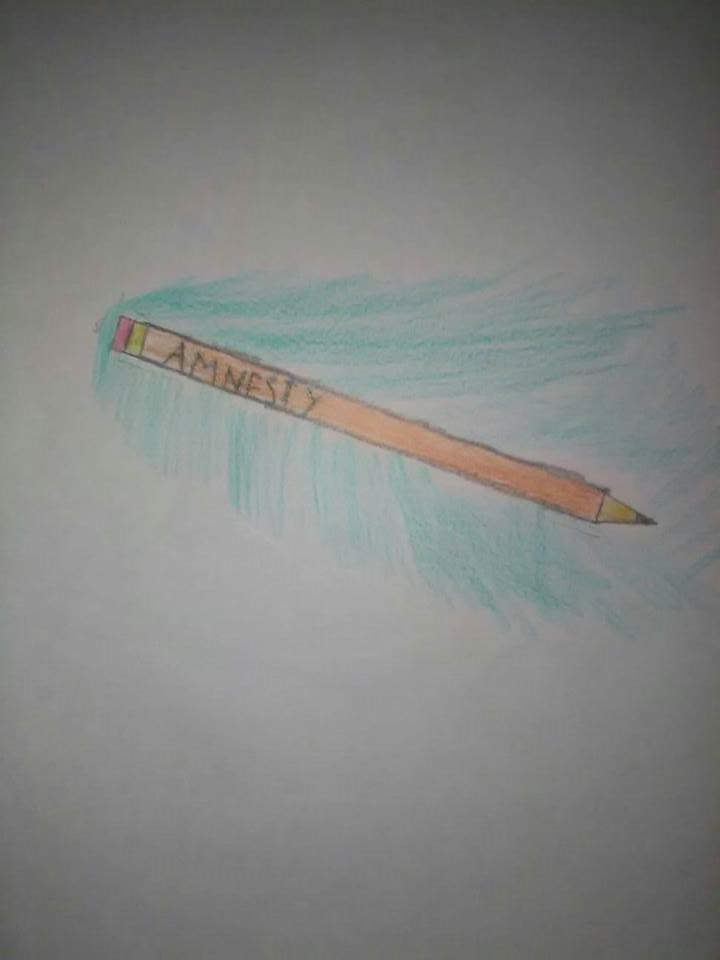The image showcases a detailed colored pencil drawing on a pristine white sheet of paper. Centrally positioned, the artwork features a standard yellow pencil, illustrated with precision and a realistic touch. The pencil is oriented horizontally, pointing towards the right. Surrounding the pencil are soft, sporadic strokes of light green and light blue, radiating outward from the pencil to give a sense of subtle motion or aura.

The top half of the pencil, near the eraser end, prominently displays the word "AMNESTY" in bold, capital letters. The pencil's traditional components are clearly visible: the pink eraser, the silver ferrule (metal ring), and the finely sharpened graphite tip. The simplicity of the background accentuates the pencil, making it the focal point of the image. The overall presentation of the artwork is clean and meticulously detailed, emphasizing both the ordinary object and the meaningful inscription on it.